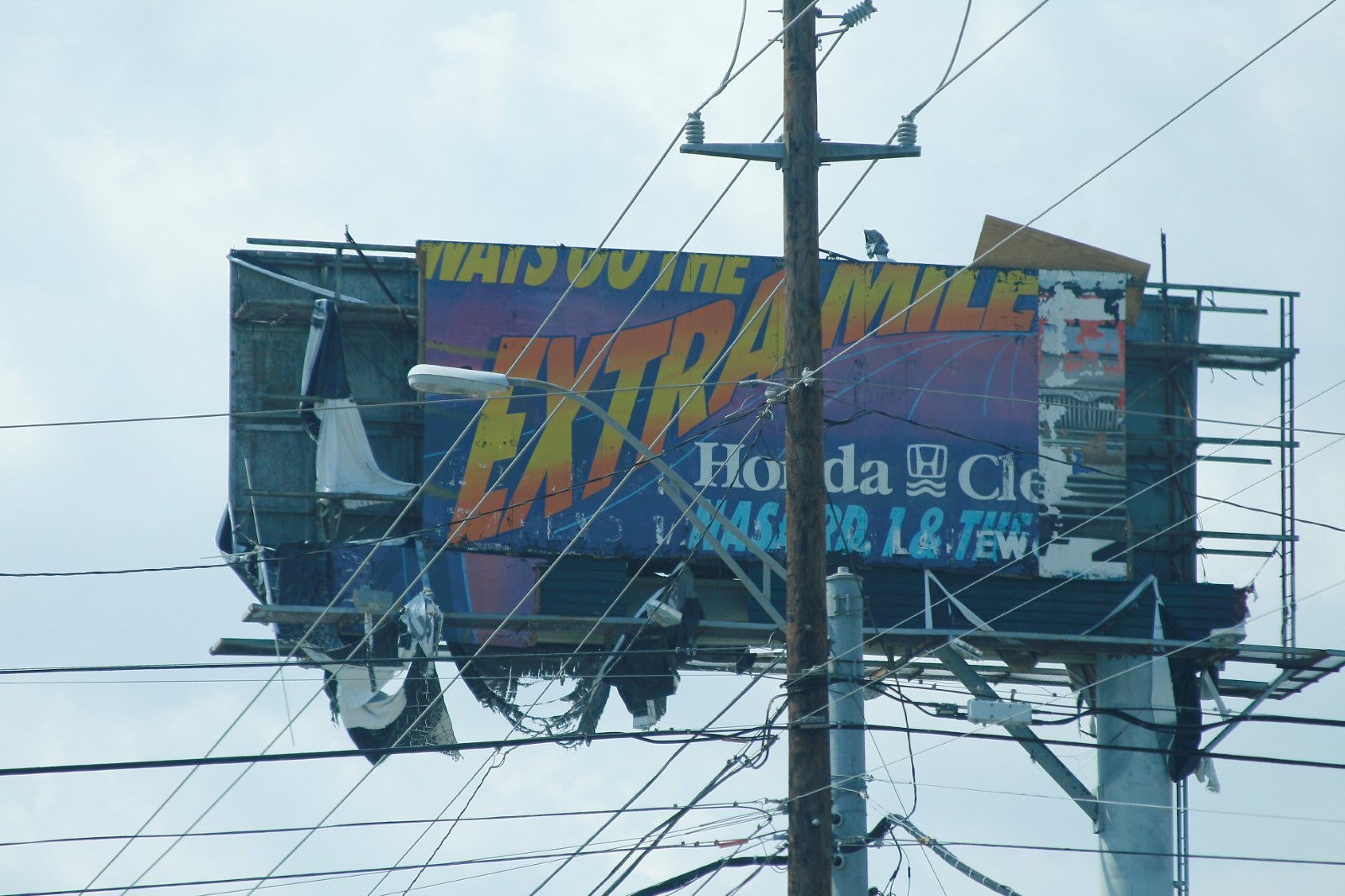In this image, we see a detailed view of a billboard obscured by several elements. A prominent brown telephone pole extends upward from the bottom to the top of the frame. Attached to the top of the pole is a silver horizontal wire. Below this wire, the main subject of the image is a square-shaped billboard sign with the words “EXTRAMILE” displayed prominently in bold orange and yellow text against a blue and purple background. Below "EXTRAMILE," the Honda logo is visible, followed by blue text. Multiple telephone wires stretch horizontally and diagonally across the frame, partially blocking the view of the billboard. The background of the image features an overcast, white-colored sky.